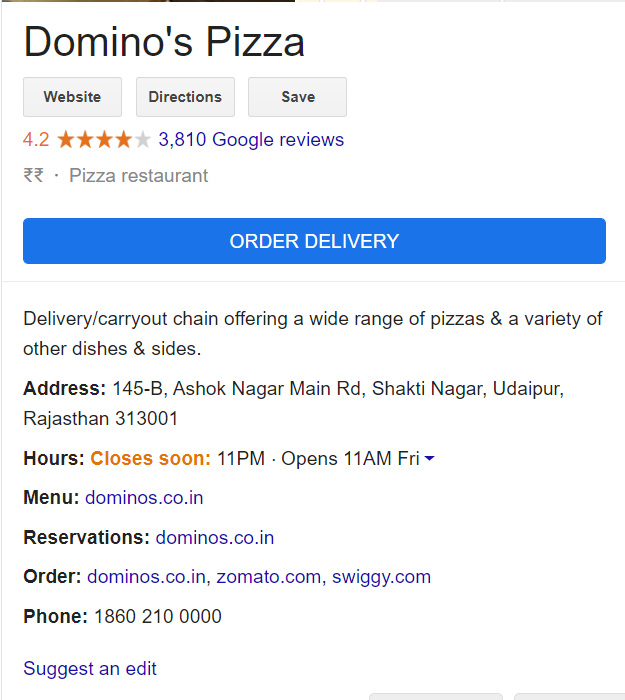The image depicts a Google search result for Domino's Pizza. At the top, "Domino's Pizza" is prominently displayed as the header. Below the header, there are three interactive options: "Website," "Directions," and "Save." A thin pixel border is seen beneath these options. The restaurant has an impressive rating of 4.2 stars based on 3,810 Google reviews. Two Indian Rupee symbols indicate that the cost is moderately expensive. To its right, it is labeled as a "Pizza Restaurant."

A large, wide, blue button is prominently featured, reading "ORDER DELIVERY" in all caps, indicating the option to place an order. Below this button, a concise description reads: "Delivery/carryout chain offering a wide range of pizzas and a variety of other dishes and sides."

The restaurant's address is provided as "145B Ashcock Nagar Main Road, Shakti Nagar, Udaipur, Rajasthan 313001." Information about the operational hours mentions it closes at 11 PM and opens at 11 AM on Fridays. There are several blue text links for the menu, reservations, and orders, all leading to dominoes.co.in. Additional ordering options are available via zomato.com and swiggy.com.

Finally, the contact number listed is "1-860-210-0000," and there is a "Suggest an edit" option at the bottom of the search result.